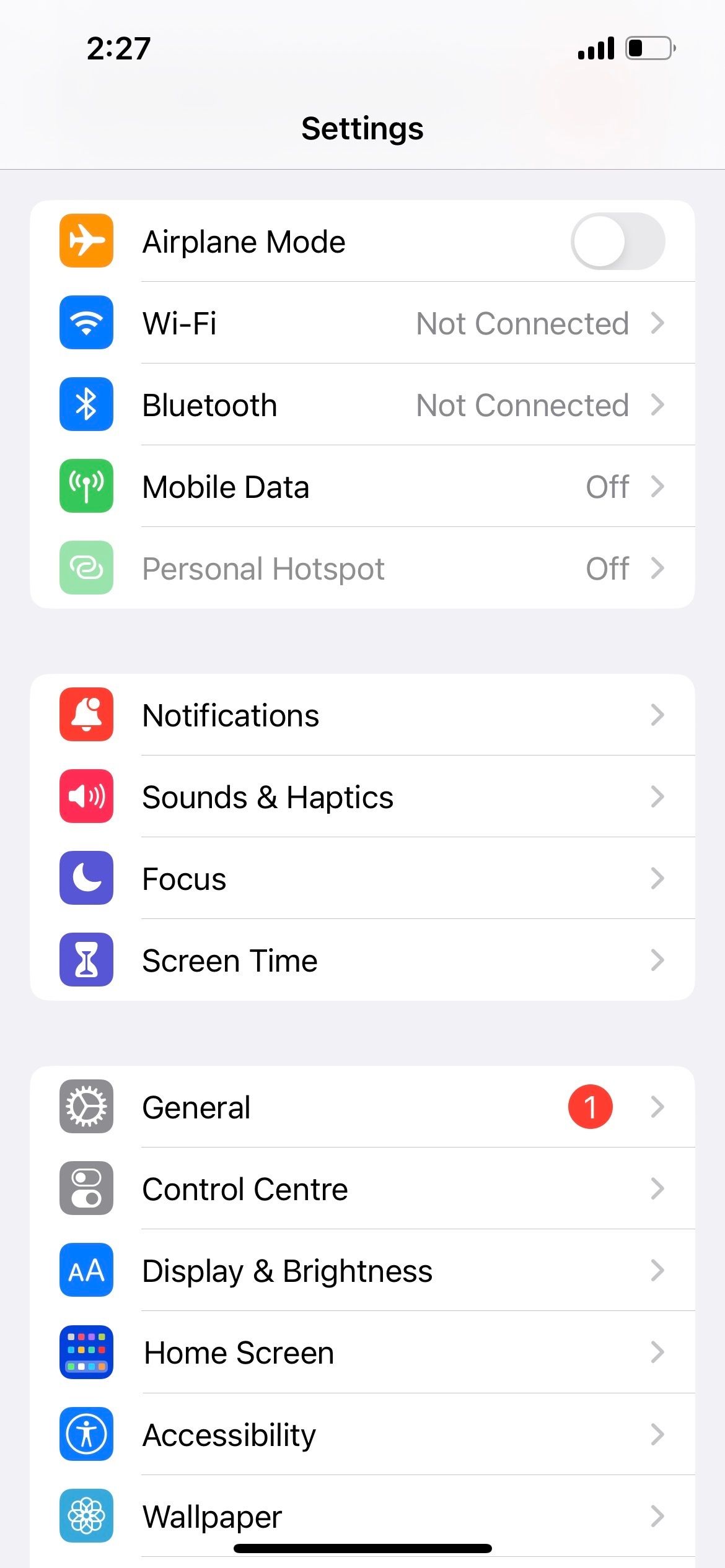### Detailed Caption

This is a screenshot of the settings page of a phone, captured at 2:27 with full 4 bars of signal strength and a battery level at approximately 30-40%. The settings page displays a variety of options, each accompanied by a colored icon on the left and a descriptive text label. The airplane mode is toggled off and represented by a white airplane icon on an orange background. The Wi-Fi option is not connected, indicated by a white Wi-Fi symbol on a blue background. Similarly, Bluetooth is not connected, represented by the Bluetooth symbol on a blue background. 

The mobile data icon, showing a beacon symbol, has a green background and is also turned off, as is the Personal Hotspot option, signified by two chain links with a light green background. Notifications are represented by a red bell icon, while Sound and Haptics is depicted by a red speaker icon. The Focus mode, identified by a moon icon, is purple. Screen Time features an hourglass icon on a purple background, demonstrating a monitoring of time spent on the device.

General settings are represented by a gray gear icon. The Control Center, displayed with sliders, also has a gray background. Display & Brightness is indicated by two capital 'A's of different sizes on a blue backdrop. Home Screen settings are signified with various small colorful icons against a blue background. Accessibility is marked by a figure with outstretched arms inside a circle, while Wallpaper settings are illustrated with a spirograph-like image on a light blue background.

Each setting is clearly outlined with distinct colors and icons, making navigation intuitive and visually guided.